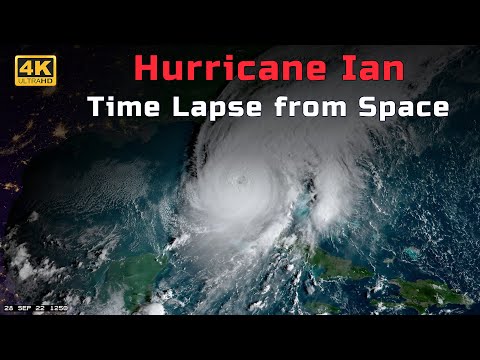The image is a high-resolution satellite photograph of Hurricane Ian taken from space, framed with black letterboxing at the top and bottom. Dominating the scene is the vibrant, white hurricane, showcasing its well-defined eye and swirling cloud formations. Below the hurricane, you can see green land formations and the blue expanse of the ocean dotted with white clouds. The vivid details highlight the clockwise rotation of the massive storm system. 

At the top of the image, the title "Hurricane Ian" is prominently displayed in bold red font, with "Time Lapse from Space" written in a crisp white font just below it. Additionally, on the upper left corner, there's a gold-bordered black square featuring the logo "4K Ultra HD" in gold lettering, signaling high-definition quality. The photograph, likely a frame from a time-lapse video, captures the awe-inspiring power and scale of the hurricane from a unique orbital perspective.